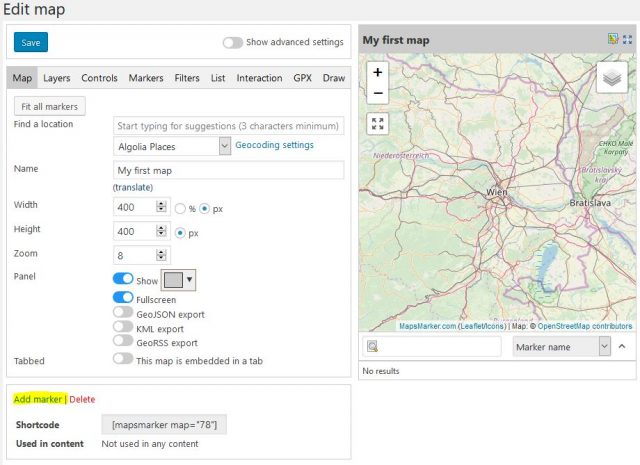The image depicts a web application's interface for editing a map. At the top left corner of the screen, a label in black text reads "Edit Map." Below this, a horizontal white bar spans the page, featuring a blue "Save" button. The bar also includes an option labeled "Show Advanced Settings," which is currently toggled off.

The interface is organized into several categories: Map, Layers, Controls, Markers, Filters, List, Intersection, GPX, and Draw. The active section is the map itself, highlighted by the command "Fit All Markers." Users can input a location and associated name in this section. Details indicate "My First Map" with dimensions of 400x400 pixels and a zoom level set to 8.

A panel displays controls that are highlighted in blue, such as "Show" and "Full Screen." There's a setting labeled "Tabbed," which is currently turned off. Below this, within a smaller section, options appear for adding a marker and deleting content. "Add Marker" is highlighted in blue with a yellow highlight, whereas "Delete" is marked in red. The section also includes a "Short Code" option intended for use within content.

On the right side of the interface, a larger map is displayed within a gray bar labeled "My First Map." The map features zoom controls with plus and minus signs. The geographical area shown includes place names in a foreign language, one of which appears to read "WIEN," and another "Bratislava."

Below the map, there's text in red and blue, along with a search bar labeled "Marker Name." Under the search bar, a message indicates "No Results."